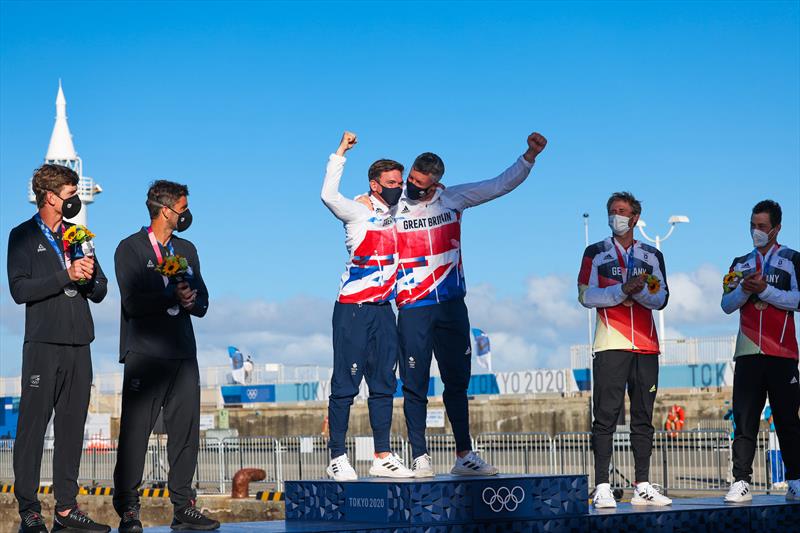In a brightly sunny, cloudless day at the Tokyo 2020 Olympic Games, a detailed image captures the award ceremony taking place inside the stadium, its walls prominently displaying "Tokyo 2020." The blue-pedestaled podium with the Olympic logo showcases six athletes proudly wearing medals. 

In the center, standing tall on the first-place podium, are two jubilant athletes from Great Britain. Dressed in white, red, and blue jerseys with "Great Britain" emblazoned on them, along with blue jogger pants and white tennis shoes with black stripes, these athletes are seen holding each other while simultaneously fist-bumping the air — the left one with his left hand and the right one with his right hand. Both are adhering to pandemic protocols by wearing black face masks.

To their left, occupying the second-place pedestal, are two somber athletes in all-black jerseys, black pants, and black face masks, holding bunches of flowers in their hands, signifying their silver medal victory.

On the right side of the podium, the third-place winners from Belgium are dressed in similar white, blue, and red jerseys paired with black pants and white tennis shoes, also donning white face masks. 

The backdrop of this celebratory moment features a stretch of grass and a fence set against the vividly blue sky, highlighting the significance of their victory and the vibrant atmosphere of the Tokyo 2020 Olympics.